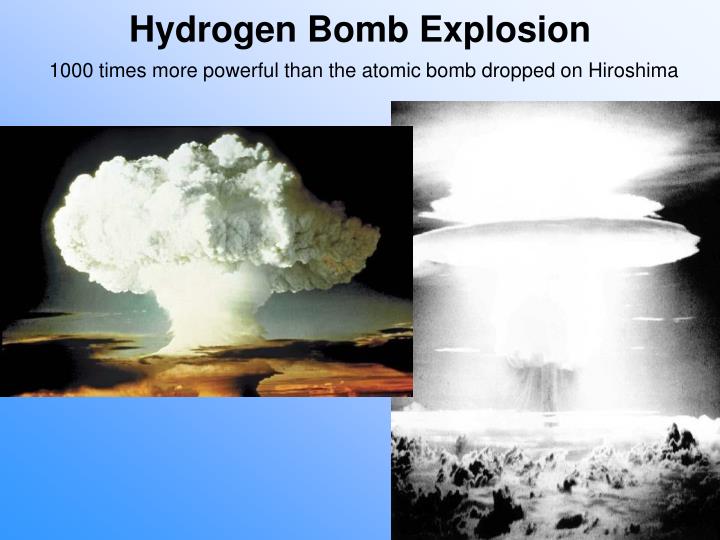The poster, titled "Hydrogen Bomb Explosion," prominently features bold black text claiming the hydrogen bomb is "1000 times more powerful than the atomic bomb dropped on Hiroshima." The background transitions smoothly from blue to white. Below the title and description lie two impactful images. On the left, a rectangular photograph in color showcases a massive mushroom-shaped cloud, its white plume rising dramatically against a brown landscape, with a dark black and light gray sky framing the powerful ascent. On the right, a square black-and-white image captures another devastating explosion, characterized by three distinct layers of bright white, disc-shaped clouds suspended in mid-air, casting radiant white rays onto a snowy terrain below. Both images serve as stark visual testaments to the overwhelming destructive power of the hydrogen bomb.